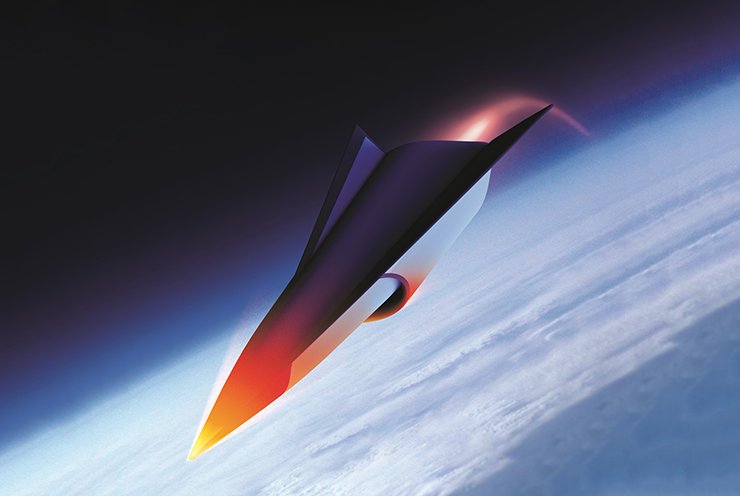This image is a computer-generated illustration of a spearhead-shaped spacecraft entering orbit, pointing diagonally towards the bottom left of the image. The spacecraft, with its sleek and smooth design, is painted in dark hues, transitioning from dark blue or purple along its body to a white bottom. The tip of the craft is intensely heating up, glowing white-hot with shades of orange, yellow, and red, creating a curved flame trail behind it. Additionally, the rear engine of the spacecraft emits a pinkish flame. The craft appears to be entering Earth's atmosphere, depicted as a vibrant blue layer gradually fading into the blackness of space, with a blanket of white clouds below. The curvature of Earth is clearly visible, emphasizing the vastness of space surrounding the scene.